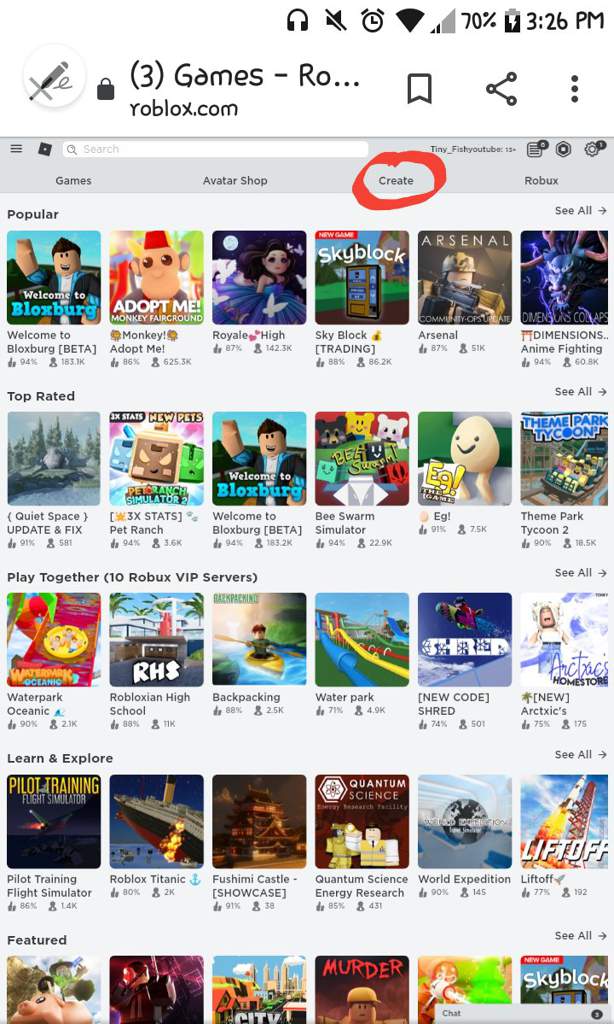This image, sourced from YoBlox.com, showcases a variety of game covers available for selection on the platform. The games are organized into several categories: Popular Games, Top-Rated Games, Play-Together Games, Learn and Explore, and Featured Games. 

At the top of the interface, users can navigate through options such as Games, Avatar Shop, Create, and Robux. The username "tiny_fishy," identifiable from YouTube, is also visible. A red circle highlights the "Create" tab, drawing attention to it.

In the Popular Games section, several games are displayed with their distinct cover art and ratings:
- **Welcome to Bloxburg Beta:** 94% rating with 183.3k likes
- **Adopt Me. Monkey Fairground:** 86% rating with 625.3k likes
- **Royale High:** 87% rating with 142.3k likes
- **Skybox:** 88% rating with 82.2k likes
- **Arsenal:** 87% rating with 51k likes
- **Anime Fighting:** 94% rating with 60.8k likes

The Top-Rated Games section features:
- **Quiet Space (Update and Fix):** 91% rating with 581 likes
- **Pet Ranch:** 94% rating with 3.6k likes
- **Welcome to Bloxburg Beta (again):** 94% rating with 183.2k likes
- **Beastworm Simulator:** 94% rating with 22.9k likes
- **Egg:** 91% rating with 7.5k likes
- **Theme Park Tycoon 2:** 90% rating with 18.5k likes

The Play-Together Games section includes:
- **Waterpark Oceanic:** 90% rating with 2.1k likes
- **Robloxian High School:** 88% rating with 11k likes
- **Backpacking:** 88% rating with 2.5k likes
- **Waterpark:** 71% rating with 4.9k likes
- **New Code Shred:** 74% rating with 501 likes
- **Arctix Home Store:** 75% rating with 175 likes

In the Learn and Explore category, the following games are listed:
- **Pilot Training Flight Simulator:** 86% rating with 1.4k likes
- **Roblox Titanic:** 80% rating with 2k likes
- **Hoshimi Castle Showcase:** 91% rating with 38 likes
- **Quantum Science Energy Research:** 85% rating with 431 likes
- **World Expedition:** 90% rating with 145 likes
- **Liftoff:** 77% rating with 192 likes

Further down, the Featured Games section displays six different game titles, although only parts of certain titles are visible. Notable mentions include a city-themed game in the third position and a murder-mystery game partially visible below it, with the final game identified as Skyblocks.

Additionally, the chat option is available at the very bottom right corner of the page, offering users a way to communicate.

This image encapsulates the diverse range of gaming experiences available on YoBlox.com, with user ratings and distinct cover art enhancing the browsing experience.